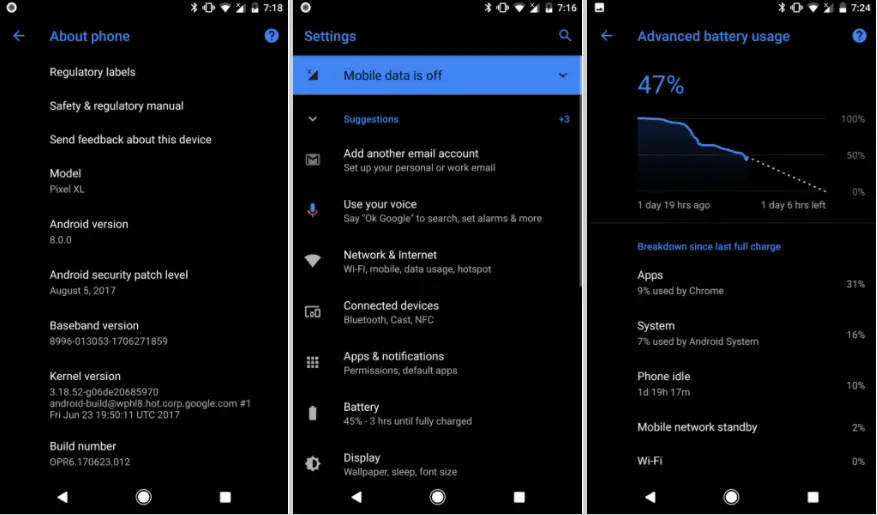**Website Screenshot Compilation**

Three side-by-side screenshots are displayed, each showcasing different settings and status screens of a Pixel XL device running Android 8.0:

1. **Device Information Screen (7:18 AM)**
   - The screen shows the "About Phone" section.
   - Battery level is below half.
   - Vibration and Bluetooth are enabled.
   - The options listed include regulatory labels, safety and regulatory manual, feedback submission, device model (Pixel XL), Android version (8), Android security patch level (August 2017), baseboard version, kernel version, and build number.
   - Navigation options featured include a back arrow and a question mark for additional information.

2. **Settings Overview (7:16 AM)**
   - The screen showcases the main Settings menu.
   - Battery level appears below half.
   - Mobile data is turned off.
   - Under "Suggestions," users are prompted to add another email account and to use voice commands.
   - Main setting categories include Network & Internet, Connected Devices, Apps & Notifications, Battery, and Display.

3. **Battery Usage Details (7:24 AM)**
   - Battery level is at 47%.
   - The advanced battery usage screen displays:
     - 9% battery consumption by Chrome.
     - 7% used by the system.
     - The phone has been idle for 1 day and 19 hours.

Each screen provides a distinct aspect of the device's configuration and usage statistics, offering a comprehensive overview for troubleshooting or informational purposes.